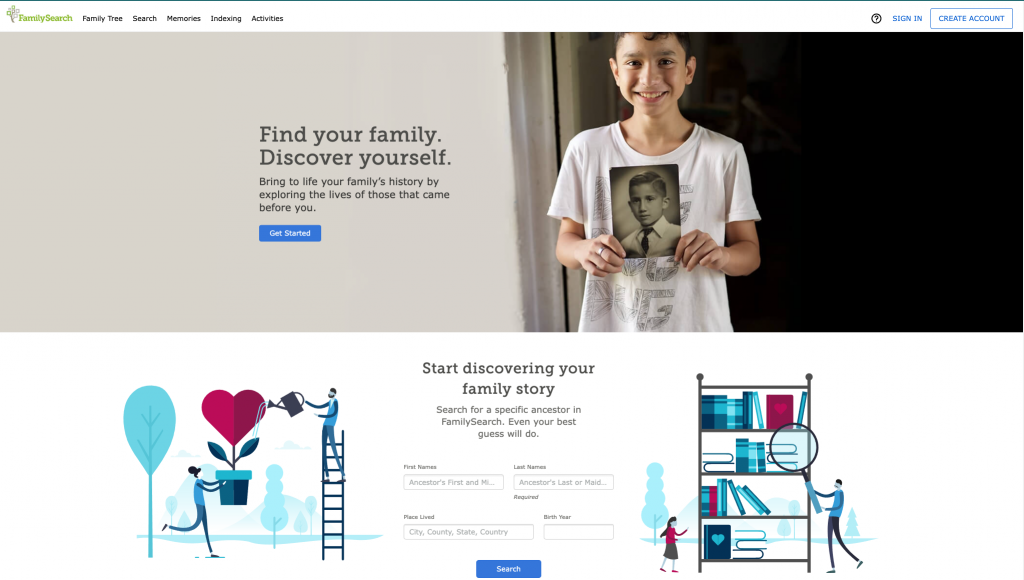The screenshot captures the homepage of the FamilySearch website. In the top left corner, the site's logo "FamilySearch" is prominently displayed. Adjacent to the logo, the navigation menu features options in black lettering: Family Tree, Search, Memories, Indexing, and Archives.

Dominating the upper section of the page, there is a large header image of a boy holding an old photograph. The boy, a white male, is seen wearing a white t-shirt and standing in a doorway. Superimposed on the image is the main headline, “Find Your Family, Discover Yourself,” followed by a subtitle, “Bring to Life Your Family's History.” Directly beneath this header is a prominent blue “Get Started” button.

The lower half of the page encourages users to “Start Discovering Your Family Story,” inviting them to search for a specific ancestor on FamilySearch. It reassures users that "Even your best guess will do." Below this prompt are four text entry boxes: the first, labeled "First Name"; the second, to the right, labeled "Last Name"; the third, placed on the bottom left, labeled "Places Lived"; and the fourth, to the right, for "Year." At the very bottom, a blue “Search” button spans the width of the entry fields, ready to initiate the search.